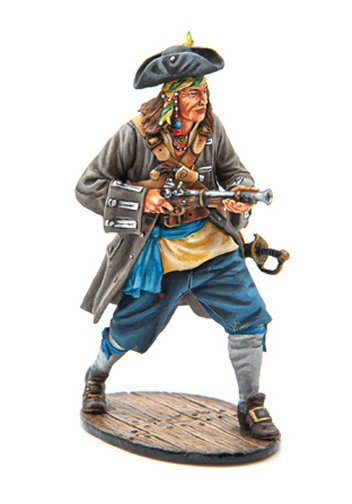The image depicts a detailed 1/6th scale figure of a pirate, who stands on a brown wooden platform. The pirate, possibly of Native American descent, sports a traditional 1800s pirate costume with vibrant elements. He wears a gray hat over a yellow and green turban and a long gray jacket with three buttons on each cuff. His outfit includes blue pants that tuck into high white socks and brown shoes with gold buckles. The figure's attire is a mix of blue, gray, and yellow tones. He holds a vintage-style gun with both hands and has a sword in a holster at his side, showcasing a blend of Native American and pirate aesthetics. The figurine's realistic and three-dimensional appearance make it hard to tell whether it is a drawing or a sculpture.